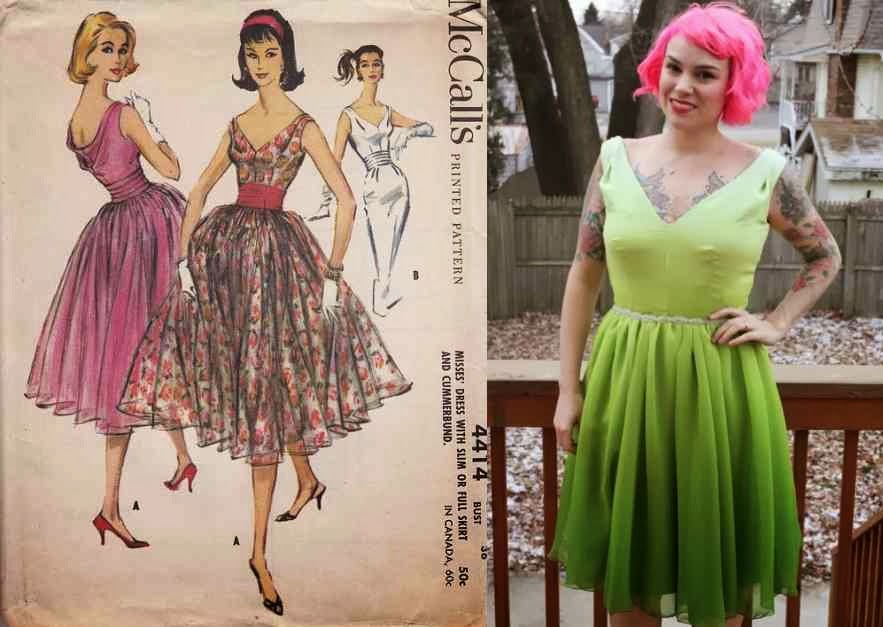The image consists of two side-by-side frames. The left frame is an illustration from McCall's Printed Pattern, showcasing three artistically rendered women in vintage dresses, marked with the pattern number 4414. Each woman is labeled with letters: A, A, and B. The first woman, positioned on the left, has golden hair, wearing a pink dress with a flowing bottom, a strapped top, and red high-heeled shoes. The middle woman dons a dress that features a red, green, and white color scheme, a red belt around her waist, and a black pair of high-heeled shoes. The third figure in the illustration, on the right, wears a full-length white evening gown paired with elbow-length white gloves. 

On the right frame, there is a photograph of a real woman standing in front of a railing. She has pink hair and tattoos on her chest and arms, and she is dressed in a knee-length green dress that transitions from light green at the top to darker green at the bottom. This woman is presumed to be the designer of the dresses depicted in the drawing.

The overall caption highlights the blend of vintage cartoon illustrations and modern fashion, linking historical dress patterns to contemporary reinterpretations.